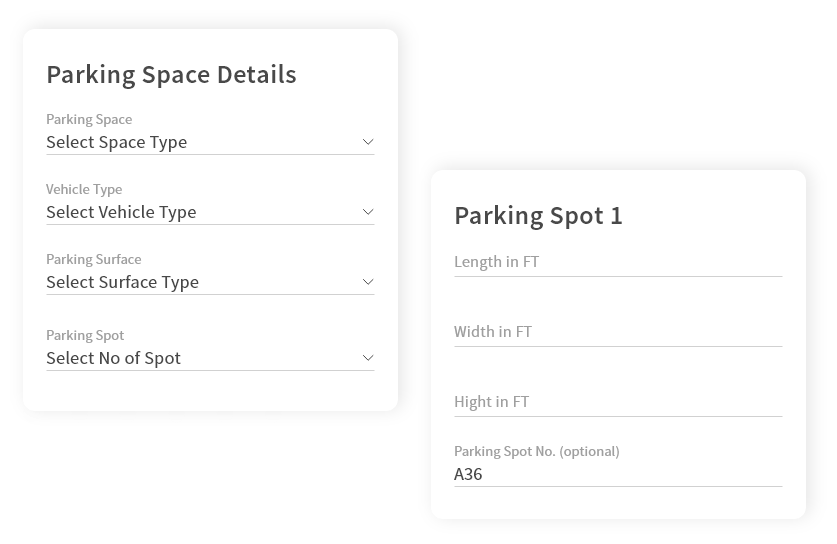The image consists of two vertical, rectangular sections with a white background and black font. Both sections are designed to provide details about parking spaces.

The first section, titled "Parking Space Details" in large black font, contains a series of grey and black text fields:
- "Parking Space" in grey font, followed by "Select Space Type" in larger black font, placed on a light gray line with a drop-down menu on the right.
- "Vehicle Type" in grey font, followed by "Select Vehicle Type" in larger black font, with a drop-down menu on the right.
- "Parking Service" in grey font, followed by "Select Surface Type" in larger black font.
- "Parking Spot" in grey font, followed by "Select No. of Spot" in larger black font, with "No." representing the number of the spot.

The second section begins slightly lower than the first and includes:
- The title "Parking Spot 1" in black font.
- Specifications for "Length," "Width," and "Height," all in capitals followed by "FT" indicating feet. Notably, "Height" is misspelled as "HIGHT."
- A field labeled "Parking Spot No." with "No." capitalized and followed by "(Optional)" in parentheses. Below this in black font is the identifier "A36."